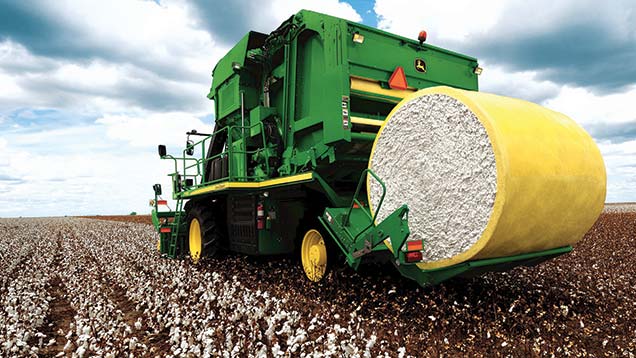The image captures a large piece of bright green John Deere farm equipment situated in a cotton field. The machine is adorned with yellow details, including its hubcaps and an orange slow-moving vehicle safety triangle at the back. The foreground of the photograph features the machinery in action, having already produced a substantial bale of cotton wrapped in yellow material, clearly visible at the front where it's being lifted. Unharvested cotton is still scattered across the field, which has a brownish hue with specks of white cotton. The expansive sky above is primarily bright blue, dotted with many white clouds casting occasional gray shadows over the scene.